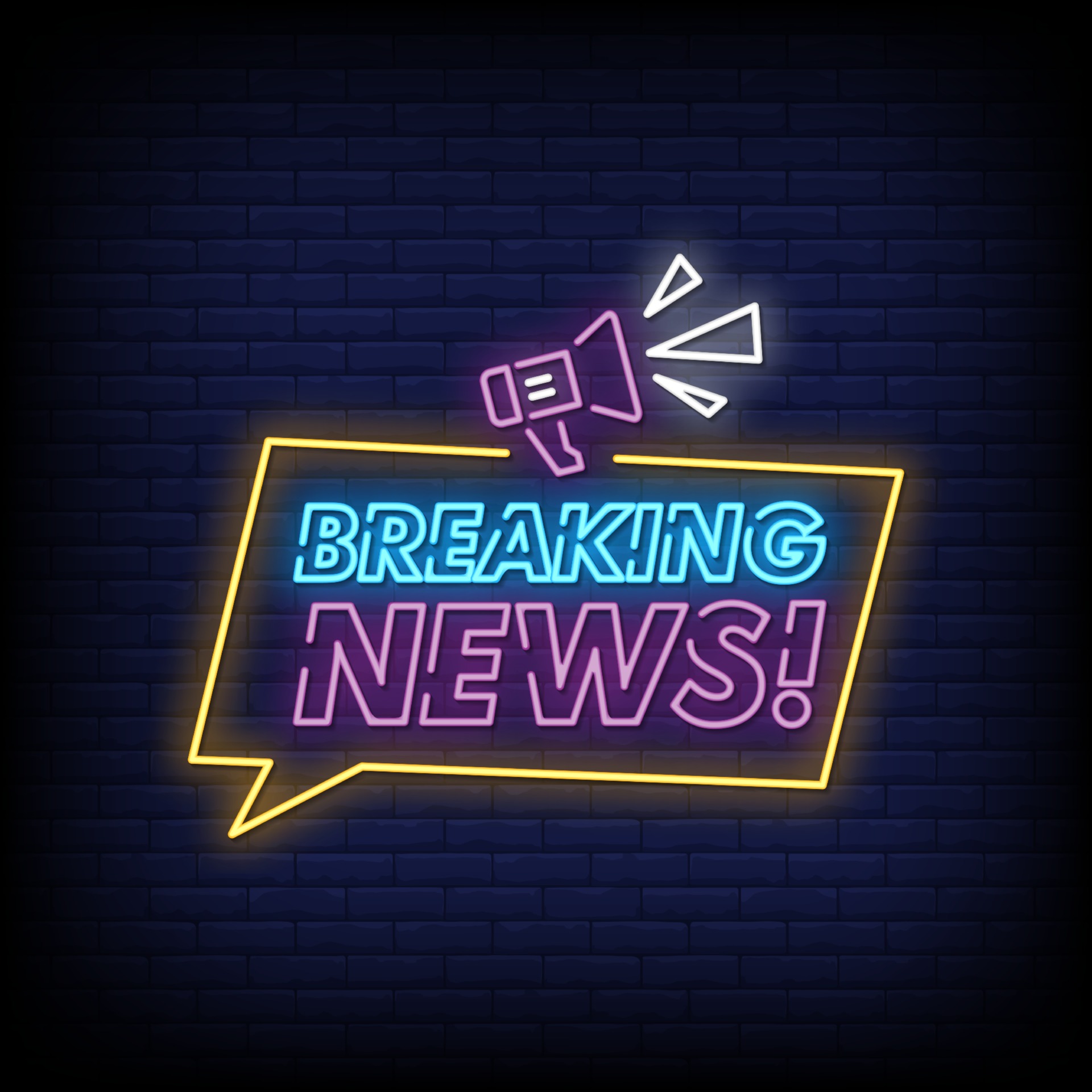The vividly designed digital image features a neon sign set against a dark blue brick wall, with the primary motif being a yellow conversation square resembling a speech bubble. Inside the square, the words "Breaking News" are prominently displayed, with "Breaking" in neon blue and "News" in neon purple. Crowning this scene, a neon purple megaphone emits white triangular shapes, signaling loudness and urgency. The overall aesthetic is dominated by neon hues, including blues, purples, and yellows, with a dark background accentuating the bright, glowing elements. This eye-catching design could serve various purposes, such as an online announcement, a digital advertisement, or a website notification for breaking news.